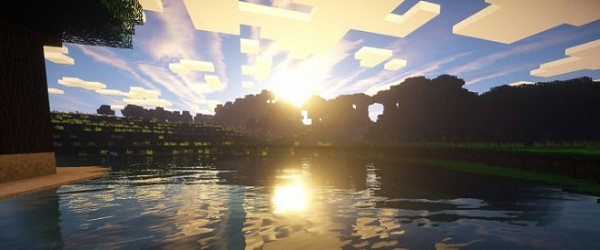This still image captures a pixelated video game scene with a tranquil and nostalgic atmosphere. At the top of the image, a bright blue sky is populated by white, pixelated clouds. Prominently, on the left side, a partly visible pixelated tree with brown bark and lush green leaves stands tall on a tan-colored base. Dominating the middle of the image is an expanse of water, rendered with surprising realism, mirroring the sun’s brilliance in the center. The sun itself is prominently positioned in the top middle of the sky, casting a gentle glow over the scene. The background boasts numerous gray mountains, which feature two noticeable openings through which the sky peeks. Nestled between these mountains and the water, several green plateaus are dotted with sparse patches of light green grass, adding depth and texture to the idyllic landscape.